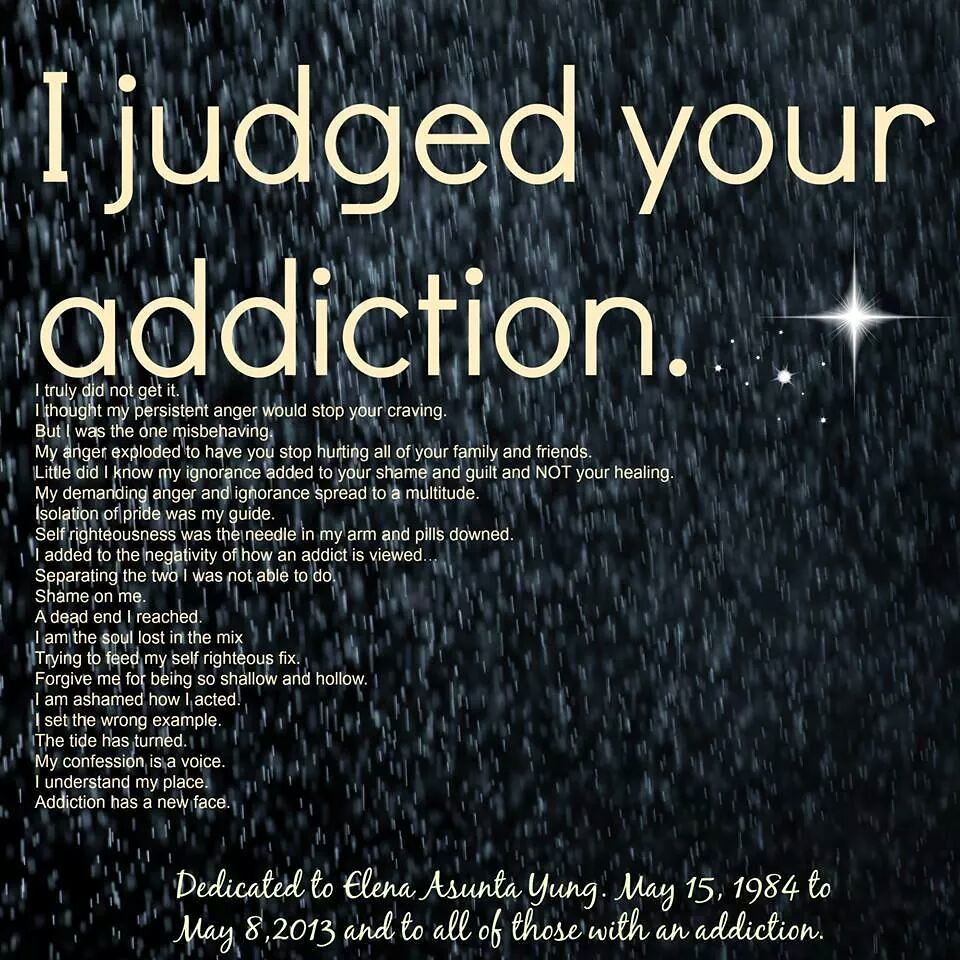This square dedication graphic features a poignant poem against a black background with delicate grayish-white lines reminiscent of rainfall, giving the image a somber tone. At the top in large cream-colored font, it declares, "I judged your addiction." To the right, a shining star subtly illuminates the scene. Beneath, the heartfelt poem unfolds, delving into the struggle of misunderstanding addiction. The finer text elaborates on the author's realization of their misplaced anger: 

"I truly did not get it. I thought my persistent anger would stop your craving, but I was the one misbehaving. My anger exploded to have you stop hurting all of your family and friends. Little did I know my ignorance added to your shame and guilt and not your healing. My demanding anger and ignorance spread to a multitude. Isolation of pride was my guide. Self-righteousness was the needle in my arm and pills down. I added to the negativity of how an addict is viewed. Separating the two I was not able to do. Shame on me, a dead end I reached. I am the soul lost in the mix, trying to feed my self-righteous fix. Forgive me for being so shallow and hollow. I am ashamed of how I acted. I set the wrong example. The tide has turned. My confession is a voice. I understand my place. Addiction has a new face."

At the bottom, a solemn dedication reads, "Dedicated to Elena Sunta Young, May 15th, 1984 to May 8th, 2013, and to all those with an addiction." This powerful graphic serves as a tribute to a lost loved one and a broader call for empathy and understanding towards those battling addiction.